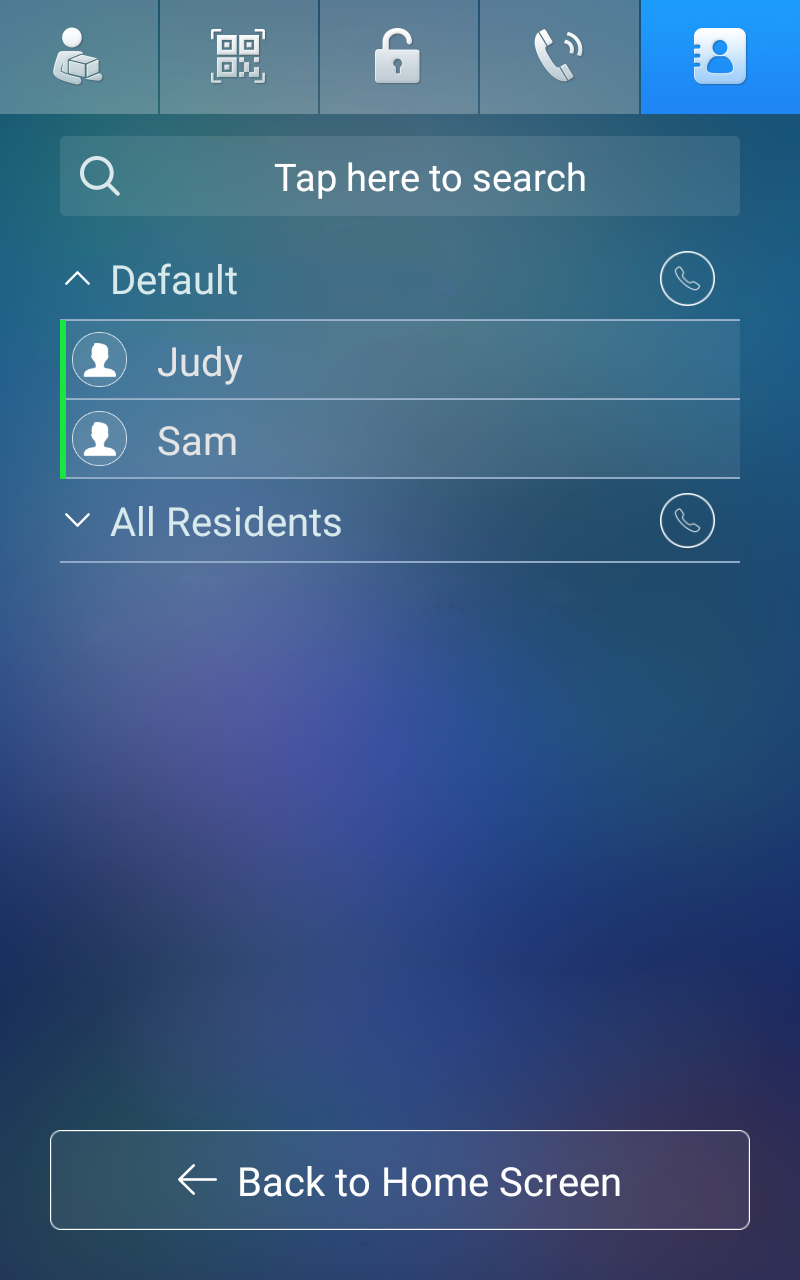This image depicts a screenshot taken from a cell phone displaying a user interface. In the top left corner of the screen, there is a cartoonish avatar of a person. Adjacent to this, there are four distinct blocks lined up horizontally. 

Below these blocks, there is an icon of an unlocked padlock, indicating that something is accessible or enabled. Following this, a telephone symbol is visible, suggesting a communication feature.

Central to the image is a blue square featuring an icon of a person. At the top of the screen, there is a search bar in the shape of a rectangle with the placeholder text "Tap here to search." 

Beneath the search bar, a section labeled "Default" is visible, followed by lines listing "Judy," "Sam," and a final option labeled "All Residents," which is accompanied by an arrow icon suggesting it is clickable.

At the very bottom of the screen, there is a button with an arrow pointing to the left, labeled "Back to Home Screen." 

The overall background of the interface is a blend of blackish navy hues with subtle touches of purple interspersed throughout.